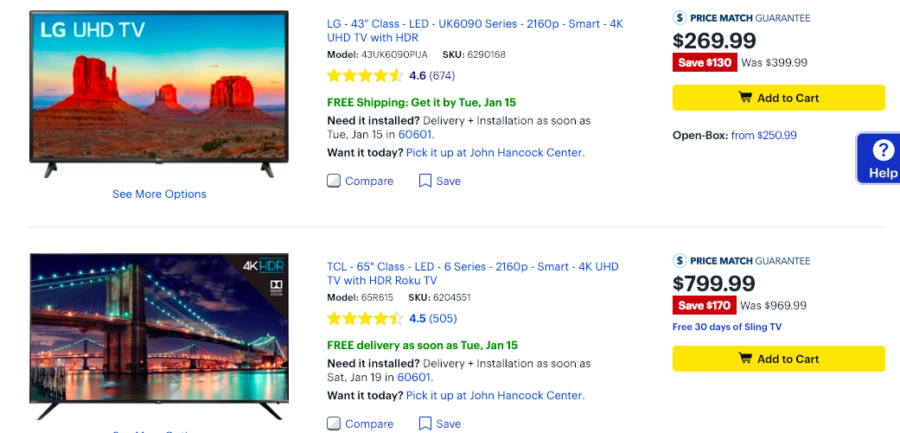The image is a detailed screenshot from a shopping website that features an LG UHD television advertised on the left side. The television screen displays a scenic image of Monument Valley in Arizona. Above the image, the text "LG UHD TV" is prominently shown, with an option to "See more options" below it. To the right, the detailed product description reads: "LG-43 inch Class LED UK6090 Series, 2160p Smart 4K UHD TV with HDR, Model 43UK6090PUA, SKU: 6290-168." The TV has a user rating of 4 out of 6 stars based on 674 reviews. Additional details mention that the item qualifies for free shipping, with an estimated delivery date of Tuesday, January 15th. There's also an option for delivery installation available by the same date within the ZIP code 60601. For those who need the TV immediately, in-store pickup is available at the John Hancock Center location. The price is listed at $269.99 after a $130 savings, originally priced at $399.99; a price match guarantee is also offered.